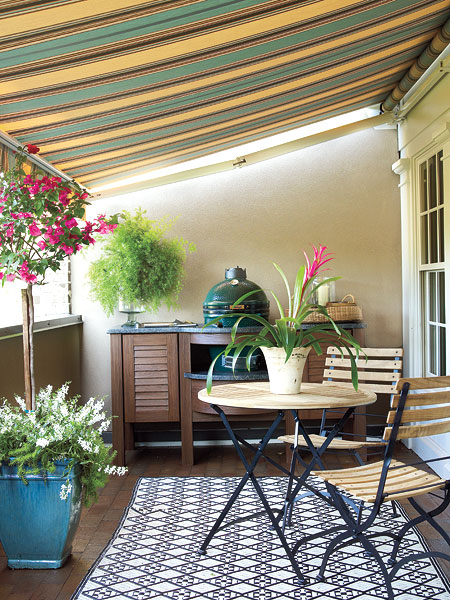This image captures a charming, cozy sunroom patio that is enclosed and designed for outdoor relaxation. The space features a small table in the center with black legs and a beige surface, surrounded by two matching outdoor chairs. On the table, there is a vibrant potted plant with lush green foliage and a striking pink flower. A navy and white area rug with a beautiful design lies underneath, defining the seating area. 

To the left of the main table is a contrasting blue table adorned with white flowers, and above it hangs a basket of blooming fuchsia flowers. The patio is shaded by a roof archway with an eye-catching striped pattern in hues of orange, red, tan, and brown, enhanced with a green and yellow valance that adds a playful touch to the décor.

In the background stands a rustic brown table or hutch holding more plants and decorations, including a small basket. Completing the space is a cabinet housing a green egg barbecue and several other garden accessories, while a door with painted glass stands to the right, offering entry to this serene retreat. The brown tile flooring adds warmth to the overall setting, suggesting a pleasant spring day with all the plants in full bloom.